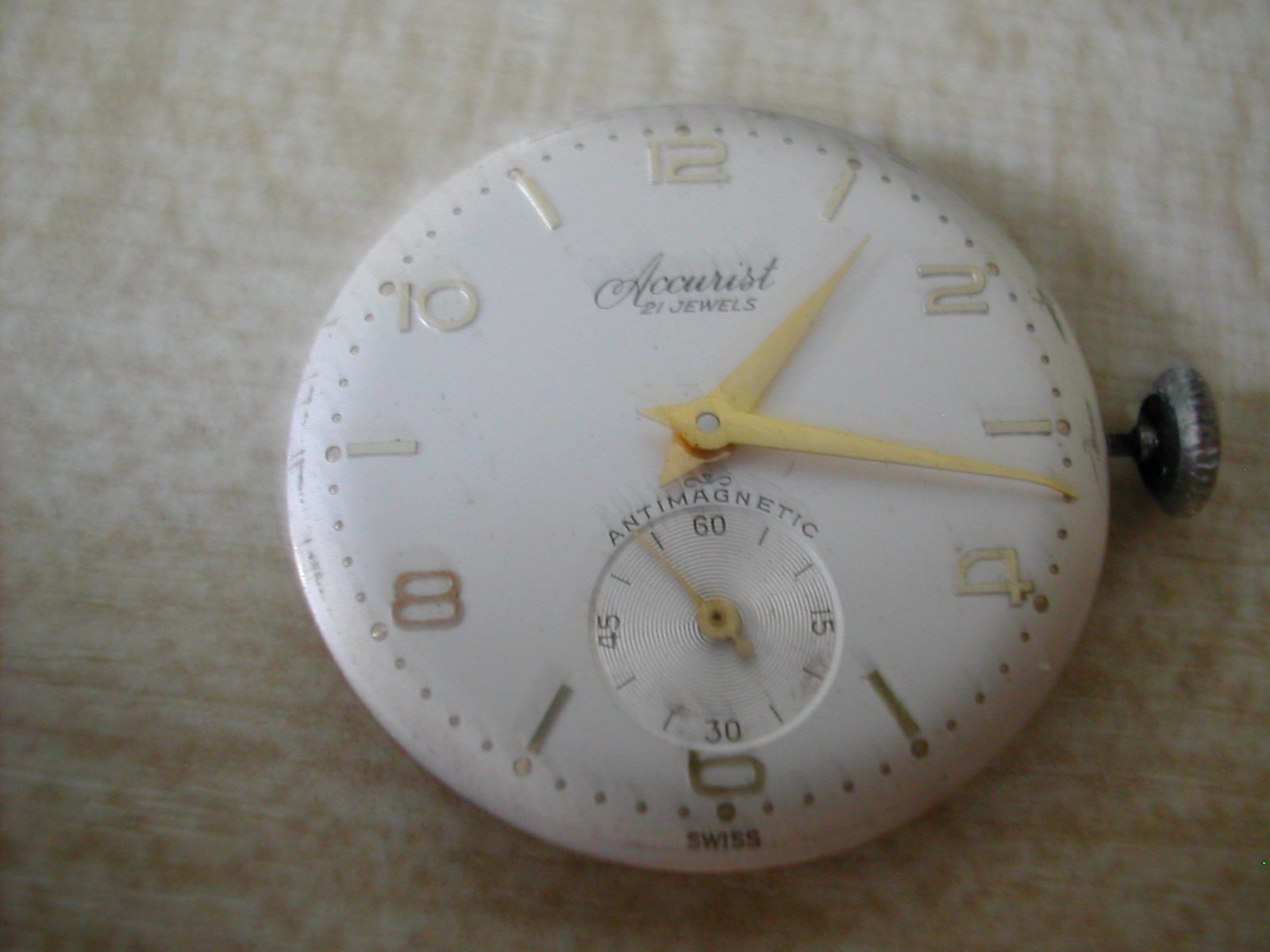The image is a realistic, horizontal photograph with a light beige, speckled background that resembles fabric or cloth. At the center of the image is a pocket watch face featuring a stopper at the 3 o'clock position, reinforcing the impression of a pocket watch without a frame. The watch face is white with gold brass hands and exhibits a unique design where only the even numbers (12, 2, 4, 6, 8, 10) are displayed in brass, while the remaining odd hours are marked by black dots. The small hand is positioned between the 1 and 2, and the large hand is between the 3 and 4. Centered on the watch face, the brand name "Accurist" and the specification "21 jewels" are printed in black text.